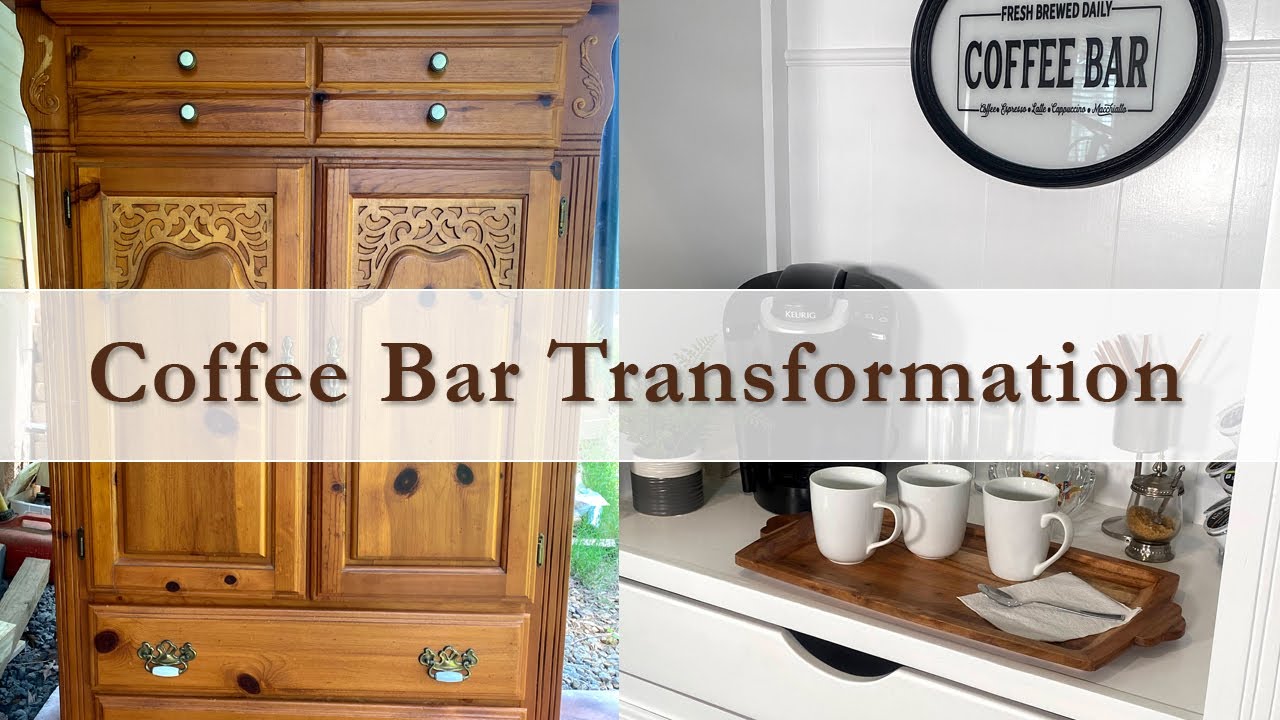The image is a horizontally-aligned rectangular composition, merging two side-by-side photographs. Across the center of the image, there's a transparent white banner that reads "Coffee Bar Transformation" in brown letters. The left photograph showcases a wooden chest with a series of drawers and cabinets featuring white round handles and brass fixtures. The chest's design includes four small drawers at the top, two rectangular cabinets with hinged doors, and two large rectangular drawers at the bottom. The right photograph depicts a coffee station setup on a white countertop with drawers underneath. The setup includes a wooden tray holding three coffee mugs, a napkin, and a spoon, alongside various coffee-making items, including a Keurig machine. Above the coffee station is a white wall with an oval-shaped sign that reads "Fresh Brewed Daily Coffee Bar" in black print on glass. Between the two areas in the center, a sliver of outdoors with visible gravel and grass can be seen. This detailed transformation highlights the evolution from a simple wooden chest to a functional and aesthetically pleasing coffee bar.